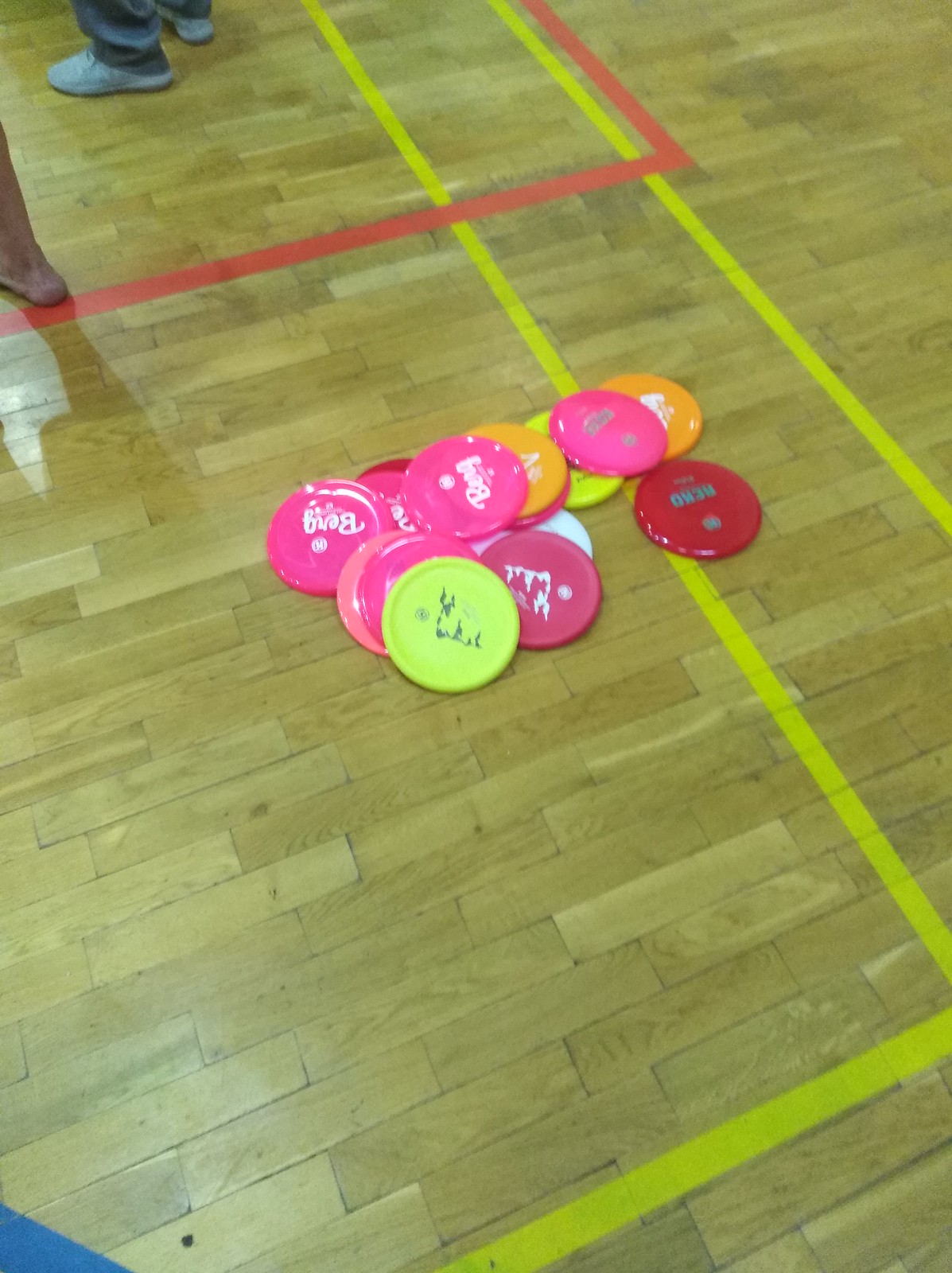This color photograph captures an indoor gymnasium scene. The smooth wooden floor of the gym is constructed from small, tightly fitted planks, with various sports lines painted on its surface—noticeably, two yellow lines forming a border and a red box within them. In the top left corner, a pair of feet in plain white running shoes appears, alongside a slightly lower bare foot, visible from the heel and casting a shadow. The middle of the image features a pile of different-colored frisbees, predominantly hot pink with faint white script logos, possibly spelling "Berg." On top of the pile lies a highlighter yellow frisbee with a black design. Other frisbees in the heap include red ones with gray prints, orange ones with similar white logos as the pink frisbees, and a single white frisbee at the bottom. Each of these frisbees remains partially obscured, making their exact designs difficult to decipher. The image has a general blurriness, likely due to a low-quality camera, but still offers a vibrant tableau of recreational equipment. Bright pink and yellow frisbees dominate the scene, standing out against the muted tones of the gym floor.